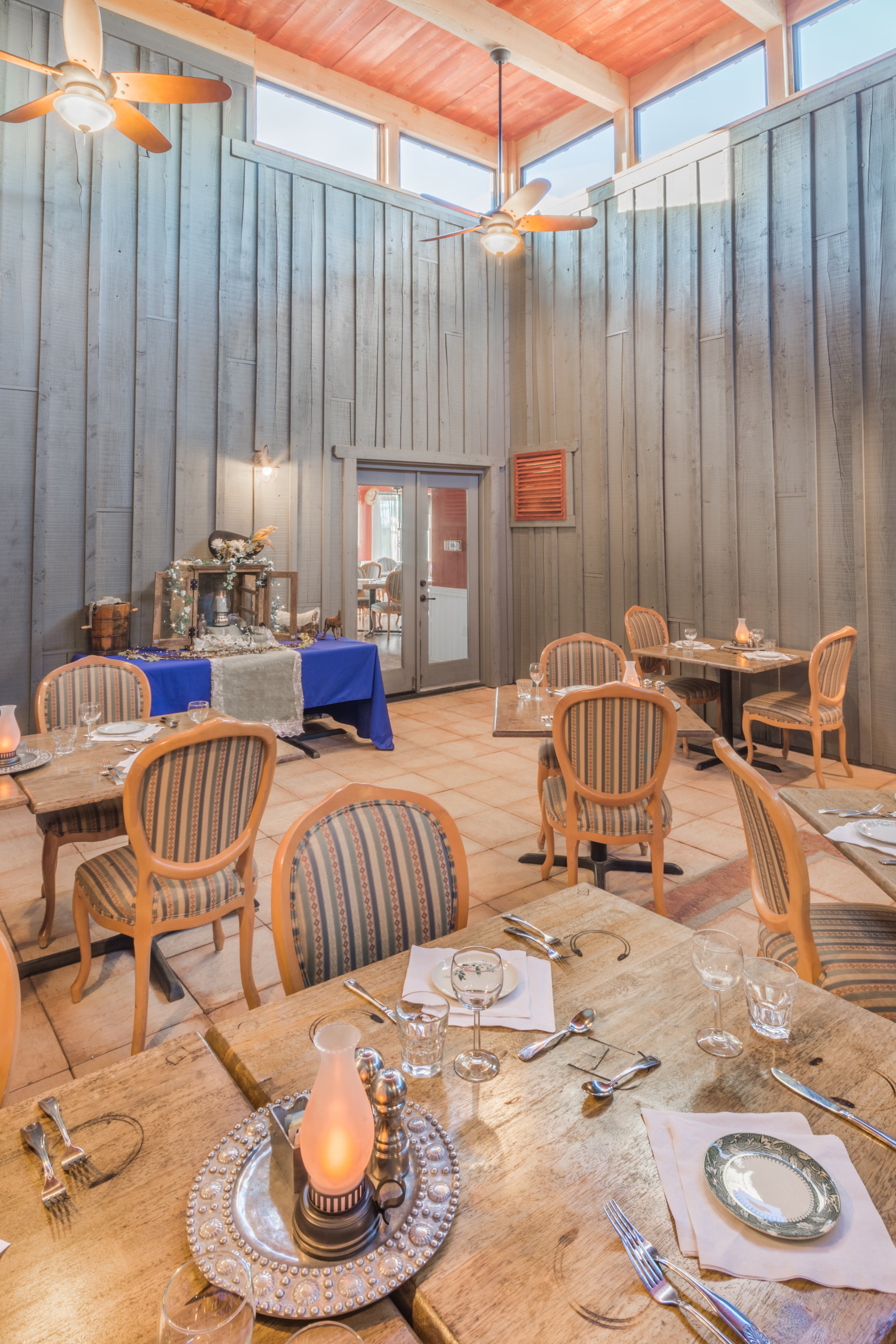This image captures the interior of a restaurant dining area designed with an elegant, luxurious farm-style theme. The restaurant features numerous wooden tables and chairs, all carefully arranged with uniform place settings that include white napkins, white and green plates, and silverware. The tables are adorned with centerpieces consisting of silver dishes holding lit pioneer-style kerosene lanterns and silver salt and pepper shakers. The dining area presents a harmonious blend of rustic charm and sophistication, with gray vertical wooden slats adorning the walls and large windows positioned at the top. The ceiling is composed of light brown wood and is supported by white wood planks from which ceiling fans hang. The tan flooring complements the natural wood tones of the tables and chairs, which mostly accommodate two diners each. In the foreground, one table distinctly features a silver plate with a lantern and additional silver items. Toward the back of the room, a larger table covered with a blue tablecloth stands next to a self-service coffee station, illustrating thoughtful design elements for convenience and aesthetic appeal. The space is well-lit by both natural light streaming through the windows and the warm glow from the characteristic lanterns.